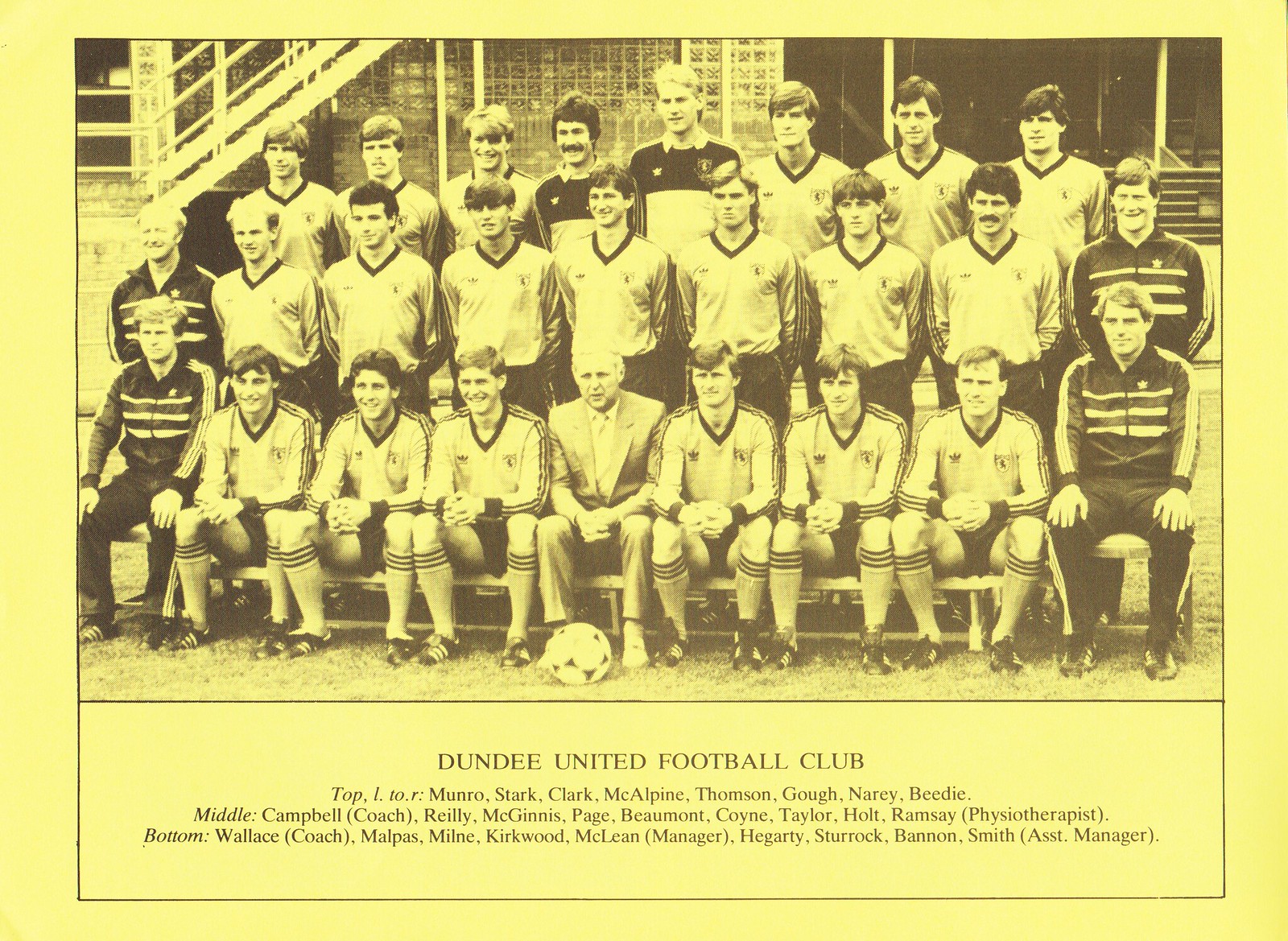This black-and-white photograph, prominently tinted in black and yellow hues, captures a formal team photo of the Dundee United Football Club, a men's team. The composition is classic of a sports team portrait, with all members aligned to face the camera. Names of the team members are inscribed in three distinct rows: top, middle, and bottom. The team members are positioned in two tiers, with some seated on a bench in the front row while others stand behind them, creating a structured formation. A white soccer ball sits centrally on the ground, symbolizing the sport. The background features a building, indicating the photo was taken outdoors, although the weather conditions are indiscernible. The expressions on the faces vary, with some subjects smiling and others maintaining neutral expressions, contributing to the authentic feel of a spontaneous team gathering.